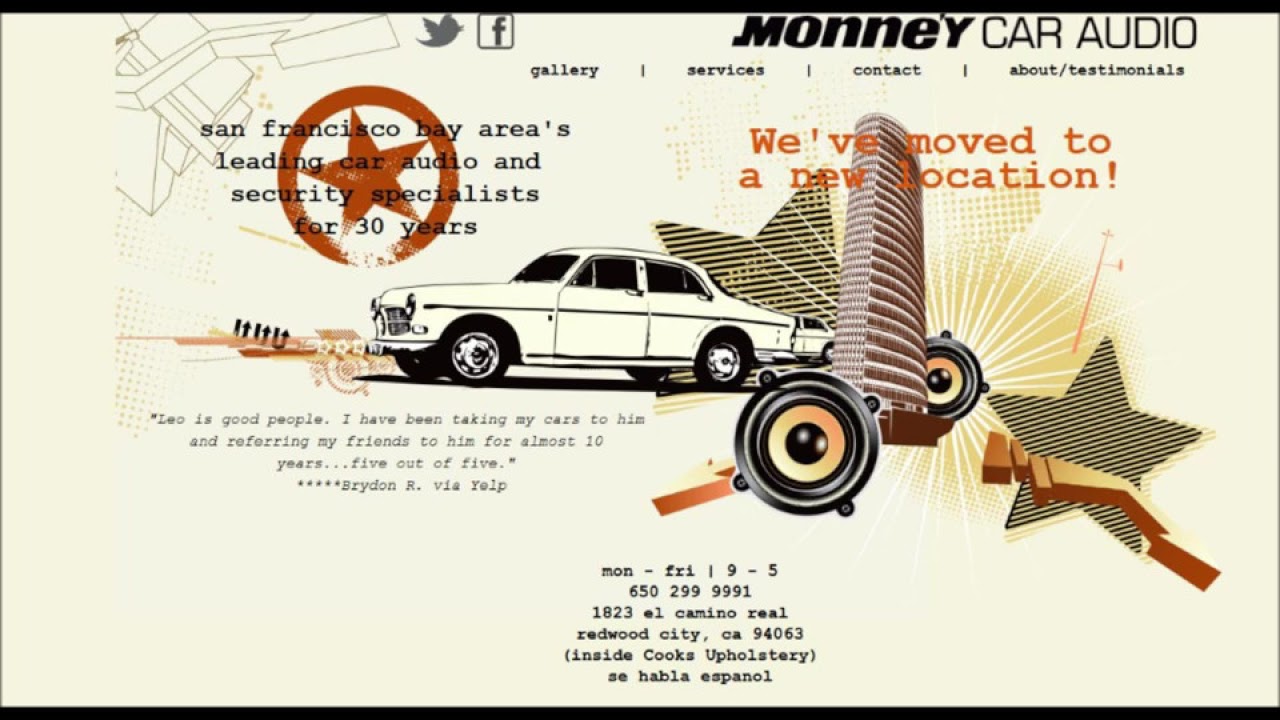This advertisement, styled similarly to a website landing page, features "Money Car Audio" prominently in the top right corner. Below the title, visitors can navigate using several options: Gallery, Services, Contact, About, and Testimonials. An orange banner announces the company's relocation. Graphically, the image is vibrant with elements like a drawn retro car, speakers, geometric shapes, stars, and social media icons for Twitter and Facebook.

Text on the left side of the image proudly states, "San Francisco Bay Area's leading car audio and security specialist for 30 years." Below this, customer testimonials are highlighted, including one from Yelp praising Leo's service over the past decade. The bottom section provides detailed contact information, including business hours (Monday through Friday, 9 AM to 5 PM), phone number (650-299-9991), and the new address: 1823 El Camino Real, Redwood City, CA 94063, inside Cook's Upholstery. Additionally, it notes "Si habla español" to indicate Spanish language support. The advertisement features a collage of cars, audio systems, buildings, and abstract art, creating a dynamic and comprehensive visual guide.